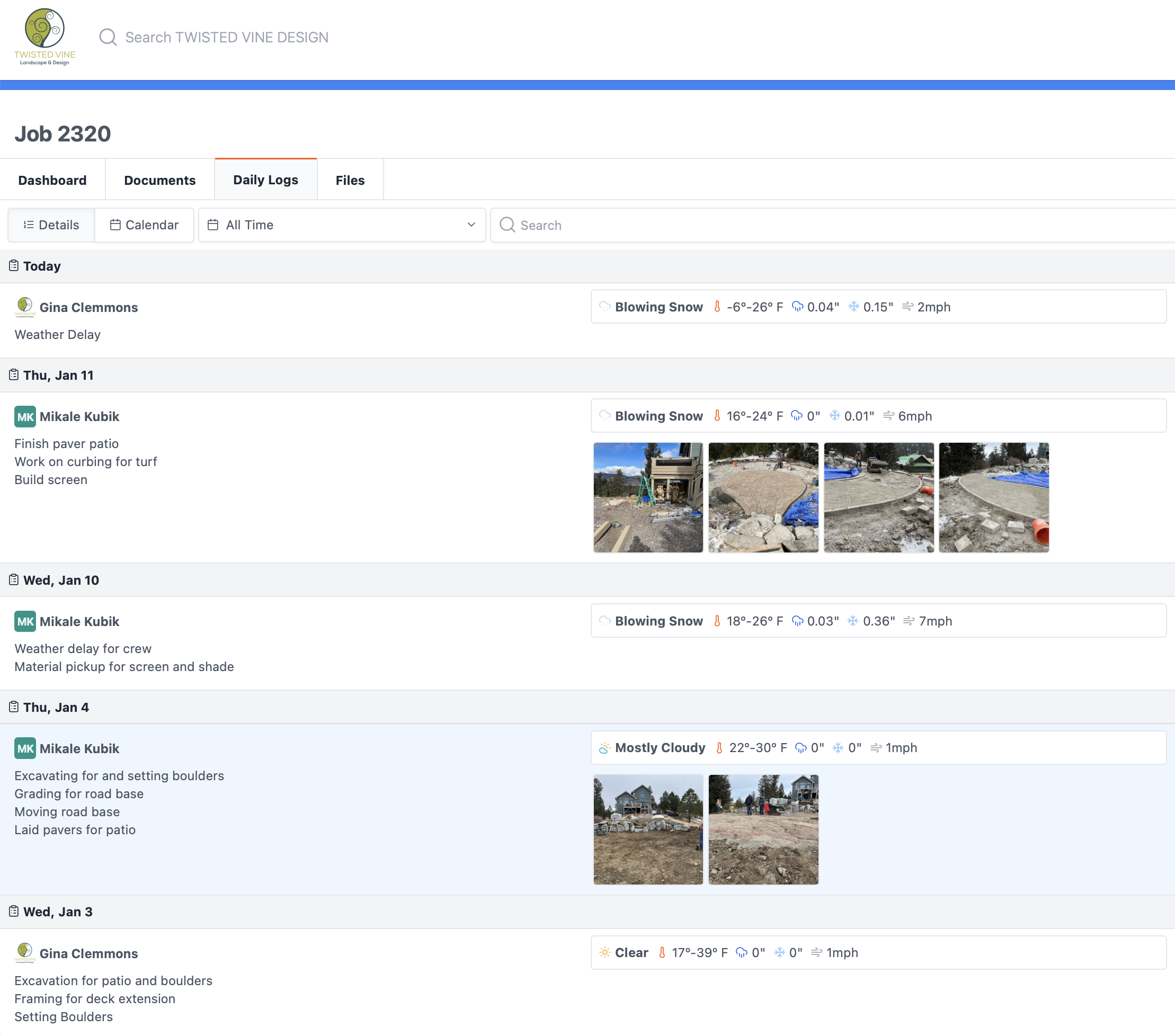**Detailed Caption for Image:**

The image depicts a clean, organized search interface set against a white background. At the top left corner, there is a green and white circular logo adjacent to a magnifying glass icon with the text "Search Twisted Vine Design". Below this is grey text, followed by a blue horizontal line. To the left, the black text reads "Job 2320". 

Underneath, there is a navigation menu in black font listing "Dashboard", "Documents", "Daily Logs", and "Files", resembling the layout of a webpage. Below this menu, grey text lists "Details", "Calendar", and "All Timed", next to a search box on the right. Directly below, today's date is labelled in black text with a calendar icon beside it.

The section following presents job entries:
- "Gina Clemens" on a weather delay noted with a green and white circular icon, indicating "Blowing Snow", temperatures ranging from 6°F to -26°F, with light snowfall of 0.04 inches, wind speed at 2 MPH.
- For Thursday, Jan 11th, Mika Kubiak is assigned to finish paving a patio and curb work for turf build and screen installation, accompanied by four images showcasing construction progress. The weather condition noted is "Blowing Snow", temperatures 16°F to -24°F, no precipitation, slight wind at 6 MPH.
- An entry for Wednesday, June 10th, features Mika Kubiak on a weather delay, tasked with material pickup for screen and shade, against a backdrop of "Blowing Snow", temperatures 18°F to -26°F, light precipitation, and wind at 7 MPH.
- For Thursday, Jan 4th, Mika Kubiak is involved in excavating and setting boulders, grading for road base, and laying pavers for a patio, illustrated with two photos of a dirt surface. The weather is mostly cloudy, temperatures range from 22°F to -30°F, no precipitation, and wind at 1 MPH.
- Finally, for Wednesday, Jan 3rd, Gina Clemons is working on patio excavation, boulder setting, and framing for a deck extension under clear weather conditions, temperatures spanning 17°F to -39°F, with no precipitation or significant wind.

This well-detailed interface provides comprehensive insights into daily logs, tasks, and weather conditions for construction management.